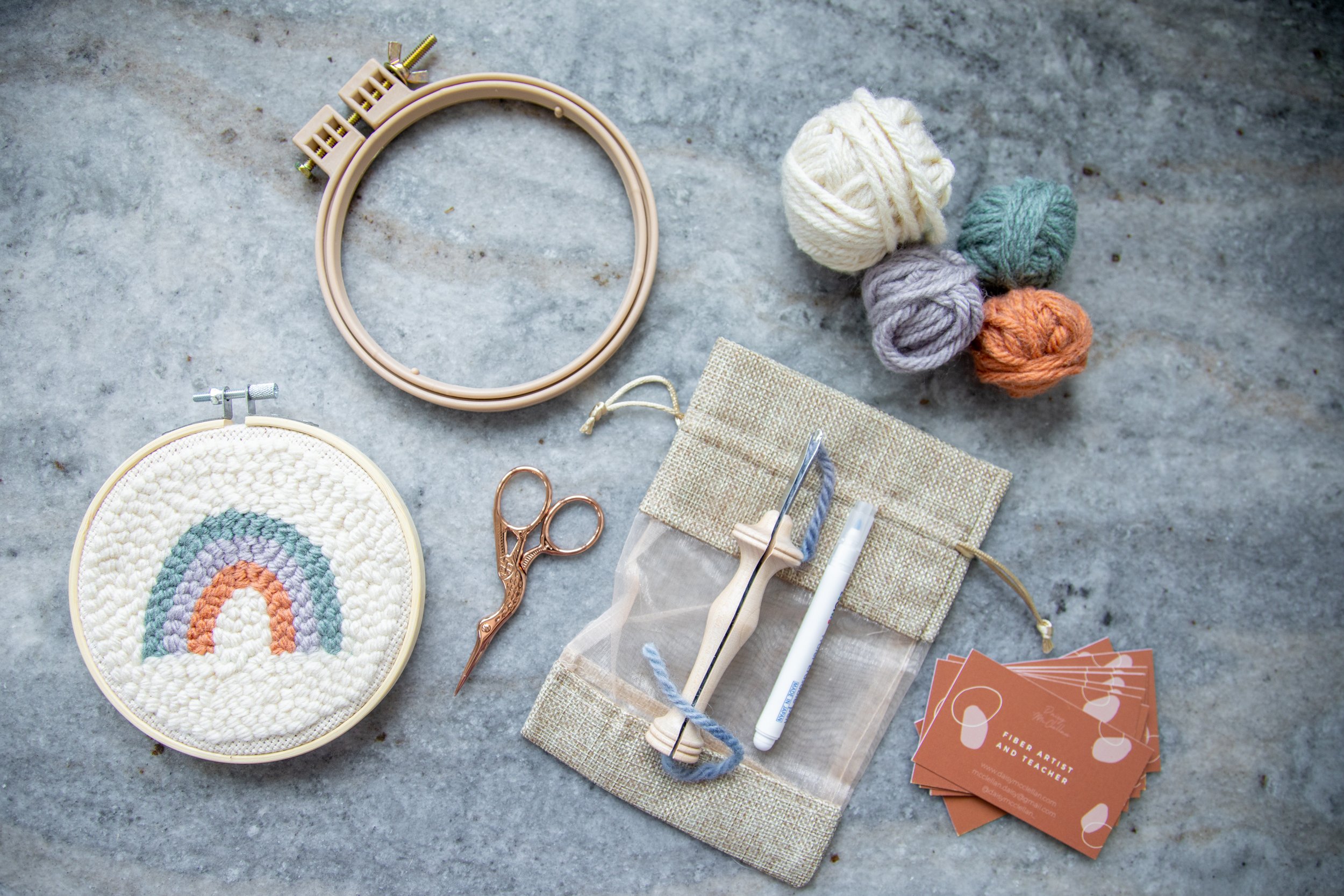The image features an assortment of embroidery and crochet tools meticulously arranged on a dark gray marble background. Dominating the bottom left is a pair of bronze or copper scissors. Positioned above, a burlap tote bag has a crochet hook resting atop it. Adjacent to this, several brown business cards are neatly placed. The upper right corner displays balls of yarn in vibrant colors: white, light purple, teal blue, and orange. Two light wooden hoops are also visible; one is empty, while the other frames a canvas depicting a rainbow that transitions from orange to light purple to teal blue on a white background. Additionally, there's a white crochet piece with a rainbow design, incorporating similar colors as the yarn. The overall composition is both orderly and visually engaging, showcasing the essentials for crafting with a harmonious blend of elements.